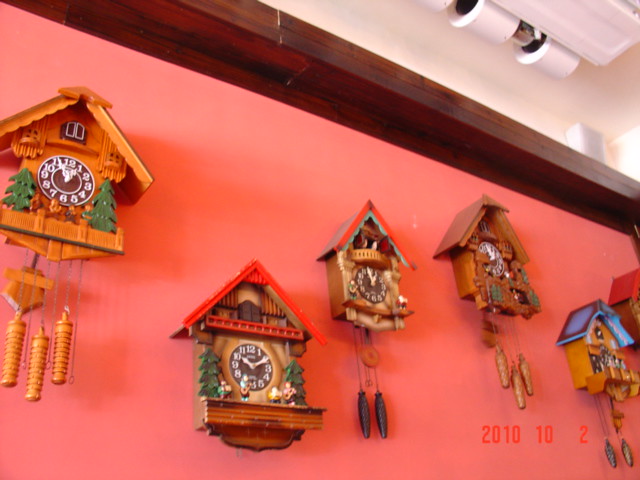In this photograph, we see a peachy coral-colored wall adorned with six cuckoo clocks, taken from a low-angle perspective as if seated near the wall. The clocks are not arranged in a straight line but vary in height along the wall. Each clock has a unique design, though all feature wooden frames. The first clock, with a medium-toned wood finish, showcases a white clock face and has three cream-colored pendulums and two green fir trees on either side of the clock face. The second clock, slightly lower on the wall, has no pendulums but also features green trees and a striking red roof. The third clock, a thinner version, has two dark brown pendulums and an orange-edged rounded balcony. The fourth clock is light brown with three pendulums and two wooden pine trees flanking its face. The fifth, identifiable by its orange railing and roof, includes three small musician figures and two counterweights. The last clock, partially seen at the edge of the frame, is yellow with a blue roof and two green counterweights, and it appears to have a porch. Above the wall, there is a wooden beam with a white material above it, possibly plastic. A date stamp, "2010-10-2," is visible in orange print on the wall.